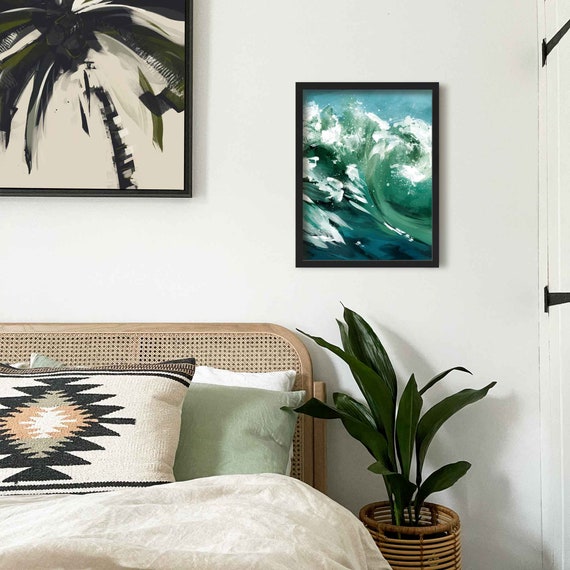This image showcases a cozy bedroom with a distinctive cane-back bed located in the lower left corner. The headboard, designed in a woven mesh style, is brown and features an array of pillows, including a white one with brown stripes and an artistic multi-pointed figure. There is also a pale green throw pillow, and the bed is adorned with a light brown to pinkish bedspread. Adjacent to the bed stands a tall green plant potted in a wicker basket.

The white walls are decorated with several pieces of framed artwork. On the right side, there is a captivating painting of the ocean with blue and green waves, evoking a sense of tranquility. To the left of this ocean scene, another piece depicts a tree, with its brown trunk and branches sprawling across the canvas. Above the bed, a black-framed, monochromatic artwork showcases a palm tree, viewed from below with its fronds hanging down. Each piece of art contributes to the serene and eclectic atmosphere of the room.